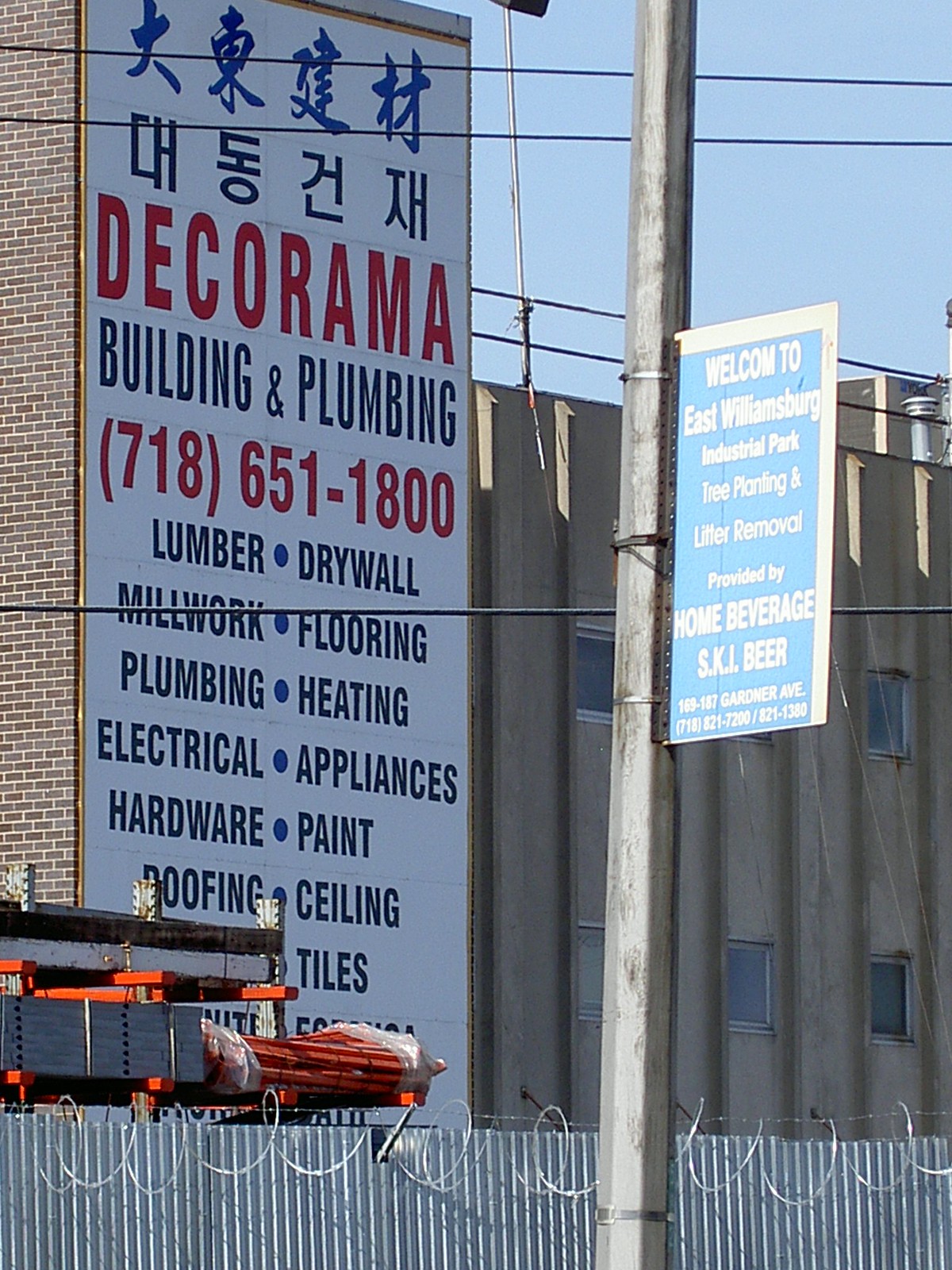The photograph captures a city street scene featuring a prominent white vertical sign on the side of a tall brick building. The sign starts with a series of oriental characters, split into two sets of four blue and black symbols respectively. Below this, in large red text, is the word "Decorama," followed by "Building and Plumbing" in black. The text in red beneath that displays the phone number "718-651-1800." The sign proceeds to list various services in black text: Lumber, Drywall, Millwork, Flooring, Plumbing, Heating, Electrical, Appliances, Hardware, Paint, Roofing, Ceiling, and Tiles. The image is clear with a striking blue sky devoid of clouds, enhanced by visible telephone pole wires. 

In the lower section of the photo, a metal fence topped with barbed wire is discernible. Additionally, a metal light pole in the foreground dons a blue sign that reads, "Welcome to East Williamsburg Industrial Park. Tree Planting and Litter Removal Provided by Home Beverage SKI Beer," followed by an address and another contact number: "169-187 Gardner Avenue, 718-821-7200 / 821-1380." The building has small windows on its right side, with a neighboring taller structure also visible.